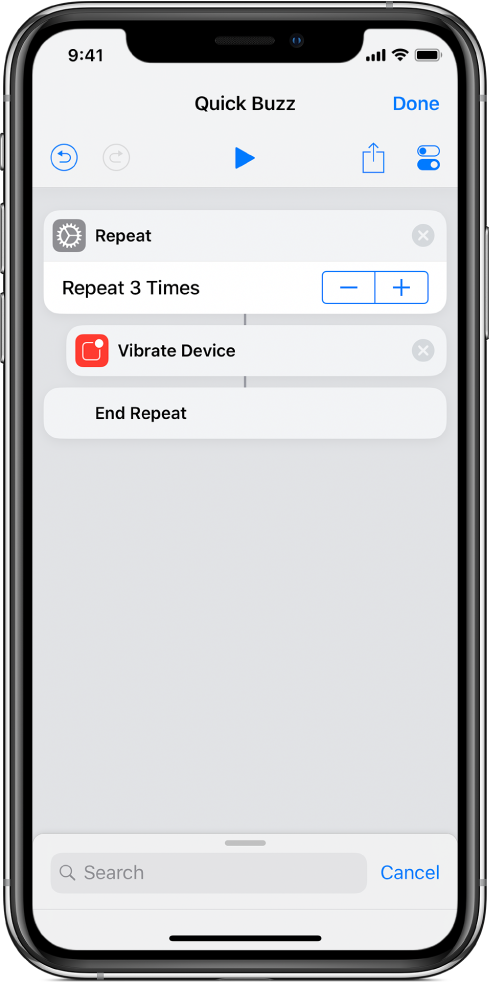The image shows a smartphone screen displaying a white page with the title "Quick Buzz" in bold black lettering at the top. To the right of the title is the word "Done" in gray text. Below the title and heading area, there are two circular icons: one is white with a blue dot in the center, and the other is blue with a white dot in the center. 

Adjacent to these circles on the left is a square icon featuring an upward-pointing arrow, indicating a download option. To the left of that is a blue triangle pointing to the right, and further to the left of that is a white circle with an arrow pointing right. Next to this is a blue circle with a triangle pointing to the left. Beneath these icons is a button labeled "Repeat" with a gear symbol next to it, white on a gray background. To its far right is an "X" symbol.

Further down, there is a section stating "Repeat three times," with a control box next to it containing a plus sign and a minus sign in blue text. Below this, a separate box labeled "Vibrate Device" appears. To the left of this box is a red button with a white square and a white circle in the upper right-hand corner of the square. To the far right of this section is another "X" symbol.

At the bottom of the screen, there is an option labeled "End Repeat" in black text. At the very bottom of the screen is a search bar with a magnifying glass icon and the word "Search" inside. To the right of this search bar is the word "Cancel" in blue text.